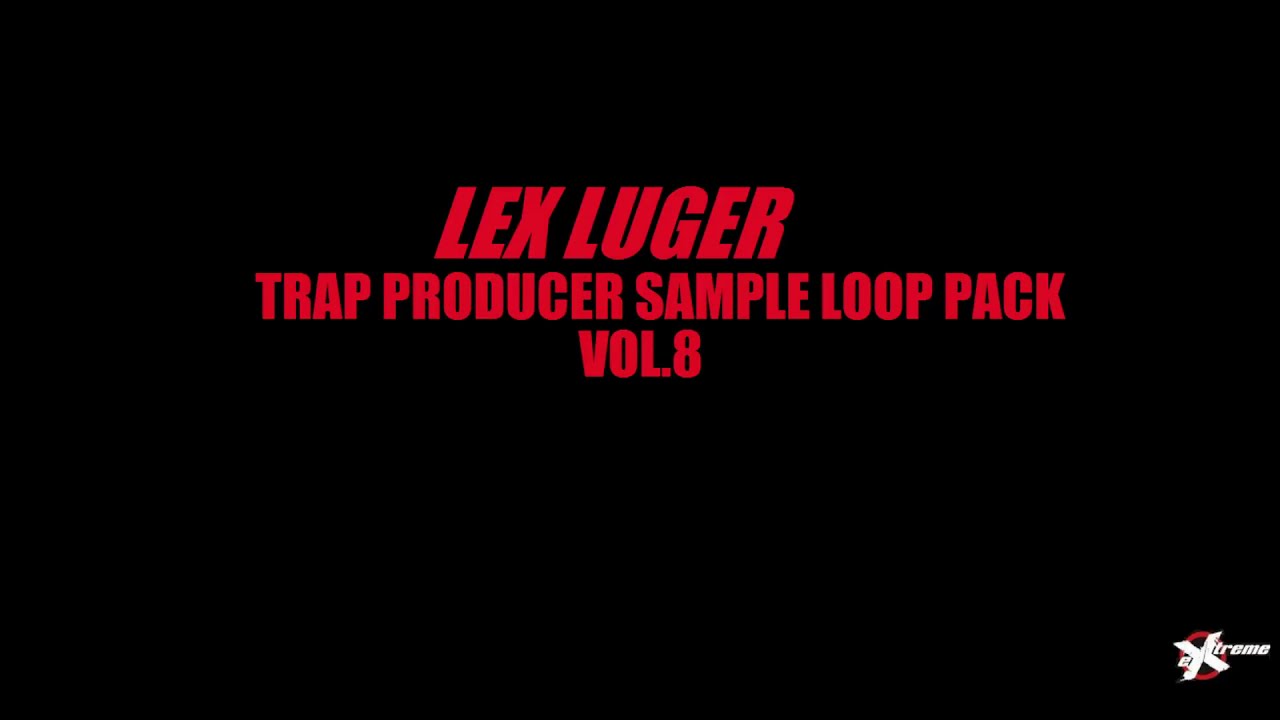The image features a solid black rectangle as the background. Dominating the center in large uppercase red letters is the text "Lex Luger," which appears italicized. Directly below this, in a slightly smaller but still prominent red print, are the words "Trap Producer Sample Loop Pack." Beneath that, in an even smaller red font, it reads "VOL 8," indicating Volume 8. In the lower right-hand corner, there's a distinctive watermark consisting of a large white X over a black background with a red circle around it. To the right of the X, the word "treme" is written in lowercase white letters, while a smaller lowercase "e" appears to the left of the X, together spelling "Xtreme." The alignment of the central text block is slightly higher than the absolute center of the rectangle but almost touching the midline.